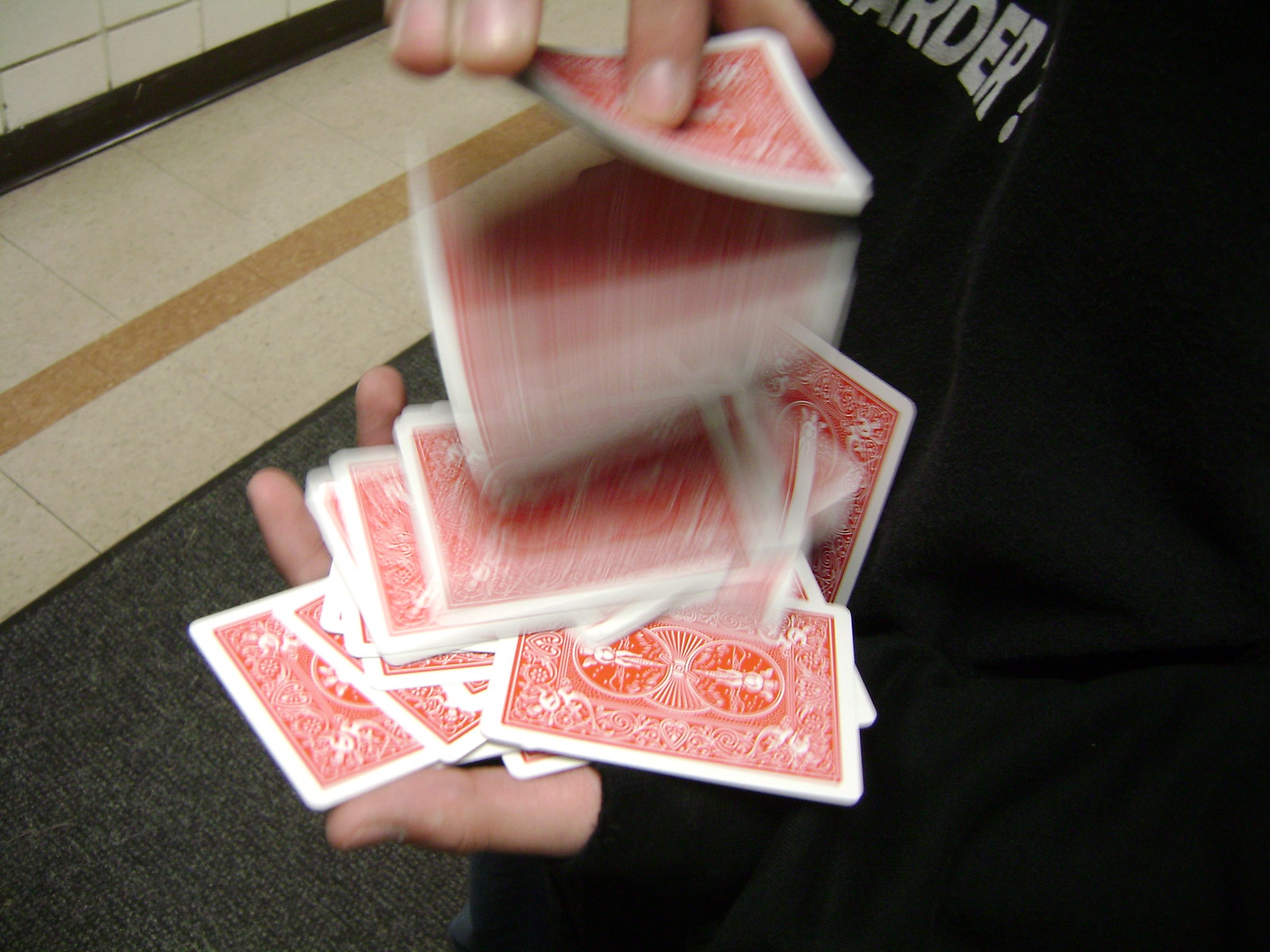The photograph captures a moment where a person is skillfully shuffling a deck of playing cards. The individual, likely a male with fair skin, wears a thick black cotton sweatshirt adorned with partial white lettering, ending in "R-D-E-R?" although the complete text is not visible due to the crop of the image. His right hand, positioned at the top of the frame with fingers pointing downward, releases a cascade of cards into his left hand, which is positioned at the bottom with the palm facing up, ready to catch them. The motion creates a beautiful blur, emphasizing the fluidity of the shuffle. Around 30 cards are visible, all with their backs facing up, displaying an intricate red and white design. The center features a dual circular motif showcasing a statuesque female figure, flanked by a radiant sun design, while the edges of the cards are bordered with an ornate, flowery pattern. The image captures the elegance and dexterity involved in the art of card shuffling.